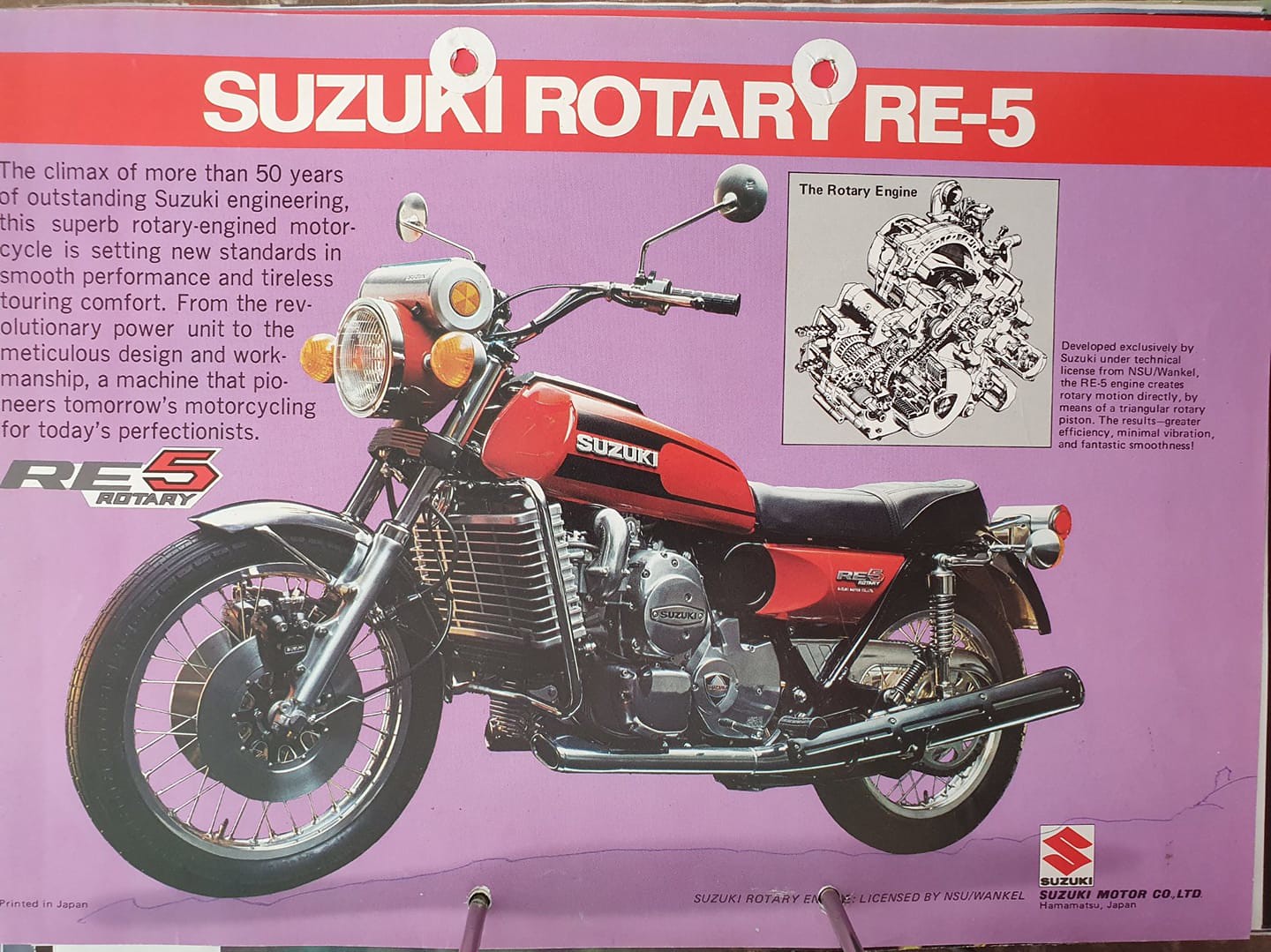This vintage advertisement for the Suzuki Rotary RE-5 motorcycle is set against a pastel soft purple backdrop. A prominent red ribbon spans the top with bold white text proclaiming "Suzuki Rotary RE-5." Below, in small black print on the left, the ad details the pinnacle of Suzuki's over 50 years of engineering excellence. The copy reads: "The climax of more than 50 years of outstanding Suzuki engineering, the superb rotary engine motorcycle is setting new standards in smooth performance and tireless touring comfort. From the revolutionary power unit to the meticulous design and workmanship, a machine that pioneers tomorrow's motorcycling for today's perfectionists."

Dominating the center of the poster is a photograph of the motorcycle itself, showcasing its striking red body and predominantly chrome structure. To the right of the image, a black and white diagram provides technical insight into the rotary engine, marked with the caption: “Developed exclusively by Suzuki under technical license from NSU Wankel. The RE-5 engine creates rotary motion directly by means of a triangular rotary piston. The result is greater efficiency, minimal vibration, and fantastic smoothness.” Completing the advertisement, the Suzuki logo is discreetly positioned at the bottom right corner.